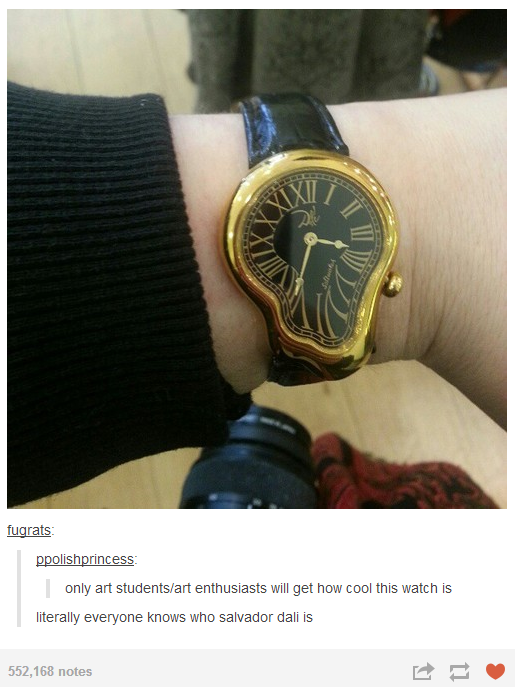The image is a close-up photograph of a unique, artistic watch adorning a person's wrist. The watch, designed with a gold bezel and a black face, features gold Roman numerals and distinct hour and minute hands. Its unusual shape captures attention; the top half is more circular while the bottom half appears warped and melting, resembling the style of Salvador Dali. The distorted face of the watch, combined with the luxurious gold elements, makes it a striking accessory. The individual wearing the watch has peachy beige skin and is dressed in a black long-sleeve shirt. They are standing on a floor with an oaky hue, partially visible in the background along with a green patterned garment. The image appears to be a post on a social media site, displaying the text: "Fugrats" and "P. Polish Princess" beneath it. It includes the caption: "Only art students and art enthusiasts will get how cool this watch is. Literally everyone knows who Salvador Dali is," and has accumulated 552,168 notes.